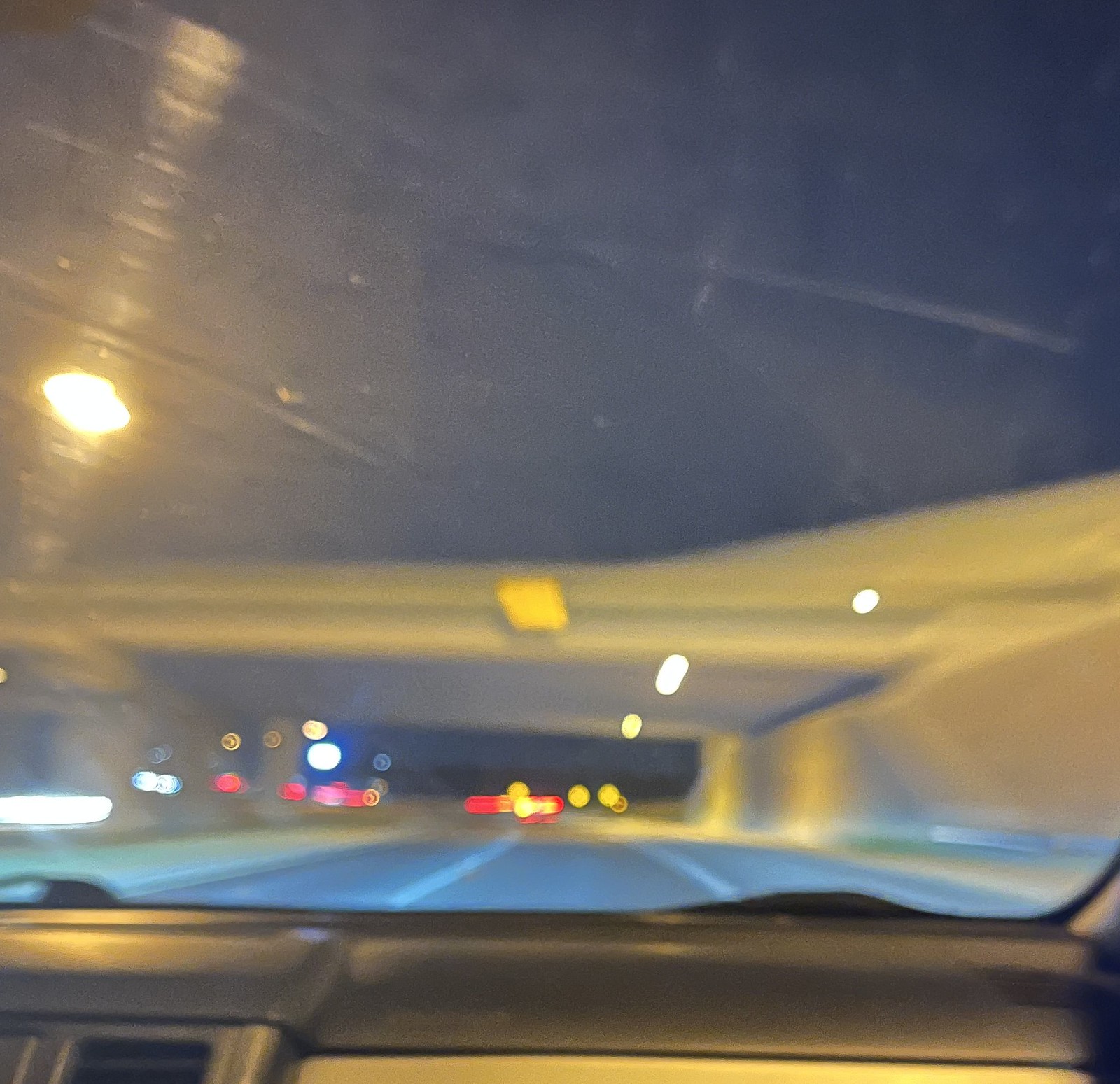The photograph captures a nighttime scene through the windshield of a car. Dominating the upper portion of the image, the sky is an inky black canvas. In the distant background, an overpass stretches across the horizon. To the left, slightly off-center, either a streetlight or the moon punctuates the darkness, casting a subtle glow. The car's dashboard spans the lower section of the image, albeit blurred, with the center console's heating duct clearly visible on the left. Farther ahead on the road, the tail lights of another vehicle can be seen, adding a splash of red to the shadowy scene.